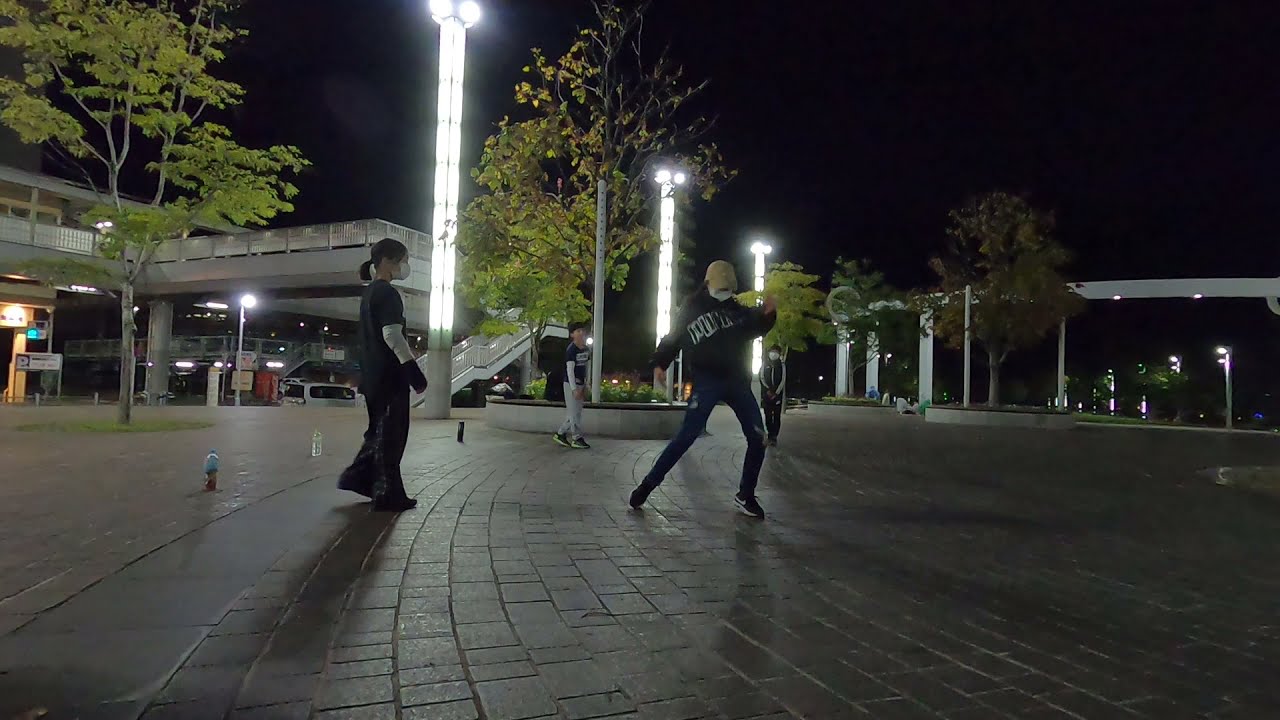The photo captures an outdoor nighttime scene in what appears to be a large, open public area with a paved stone-brick surface. The setting resembles a town center or an industrial area, possibly near a transit hub such as a train or bus station, or maybe even an airport. To the left, a multi-level parking structure can be seen, illuminated by scattered light poles. On the right, there is a smaller lit structure, the details of which are unclear, but it could be a monument or a monorail track.

In the foreground, four people are gathered, seemingly engaging in a playful activity or dance. They are dressed in dark clothing, mostly navy blue and white, and are wearing masks. One of the dancers stands out with a yellow cap. Behind them, there are shadows of additional onlookers in the background, possibly participating or simply watching the activity unfold. Surrounding the area, a catwalk with stairs and railings can be seen, along with a tree with green leaves. The scene is vividly lit by numerous light poles, enhancing the nighttime ambiance.